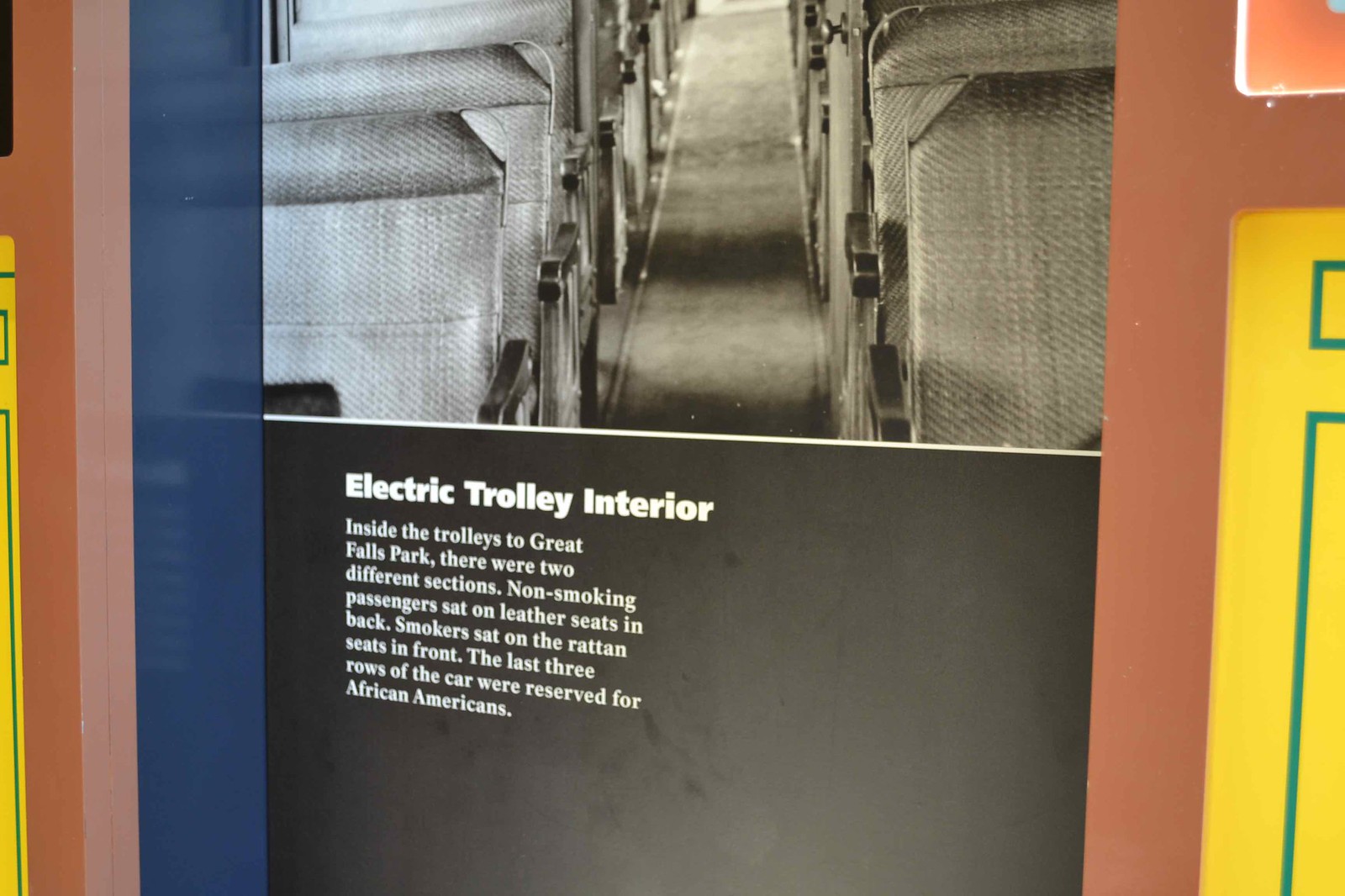The photograph depicts a museum display featuring a black and white banner on a colored wall. The banner presents an image of the aisle inside a trolley, with seats visible on both sides leading towards a distant point. The upper half of the banner shows the interior of the trolley, likely a corridor from a train or bus, detailed with rows of chairs. Stripes from the wall on either side of the banner suggest slight distortion in the framing of the photo. Below the image, a text section includes a title and a descriptive paragraph. The title reads, "Electric Trolley Interior," and the paragraph explains the seating arrangements within the trolleys to Great Falls Park: non-smoking passengers sat on leather seats at the back, smokers occupied the rattan seats in the front, and the last three rows were designated for African Americans. This detailed setup implies the display is part of an exhibit, highlighting historical social segregation within public transportation.